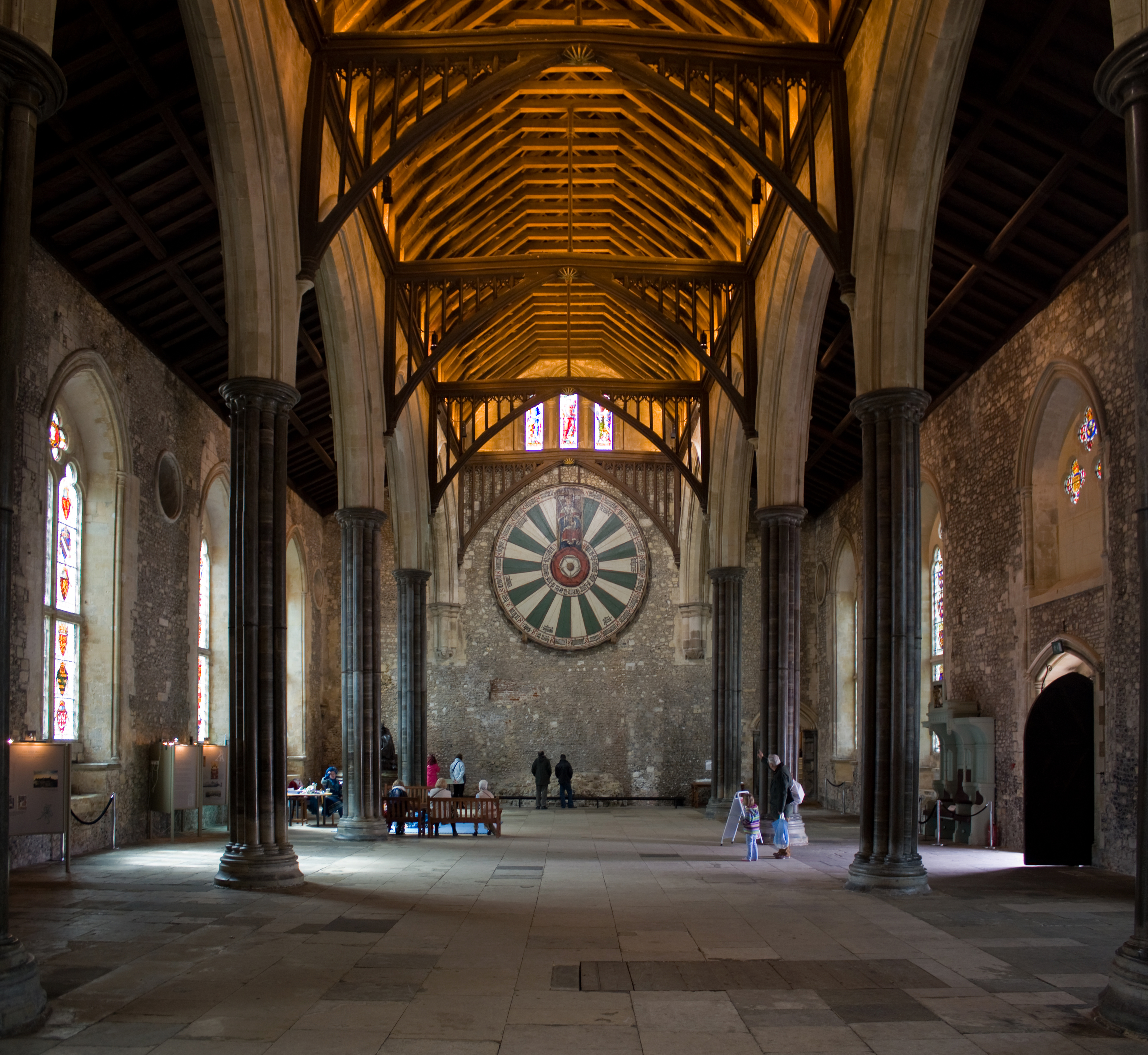This image captures the interior of an expansive, cathedral-like structure. The architecture features a sprawling tile floor, suggesting a historic or majestic ambiance. Overhead, the ceiling is adorned with wooden trusses and beams, adding an intricate and lofty touch to the structure. Soaring stone columns line both sides, supporting graceful archways and a series of large windows endowed with stained glass, which filter colorful light into the space.

The focal point of the image is a prominent brick wall at the far end, showcasing a grand circular design with alternating green and off-white tile segments that converge toward a red center, resembling a dartboard. Above this circular design are three elongated stained glass windows offering a regal, multi-colored glow.

Adding life to this historical scene, people are seen moving throughout the space—some walking, others seated at tables and benches scattered around. The overall atmosphere is one of grandeur and historical reverence, with each architectural element combining to create a visually mesmerizing and detailed interior view.